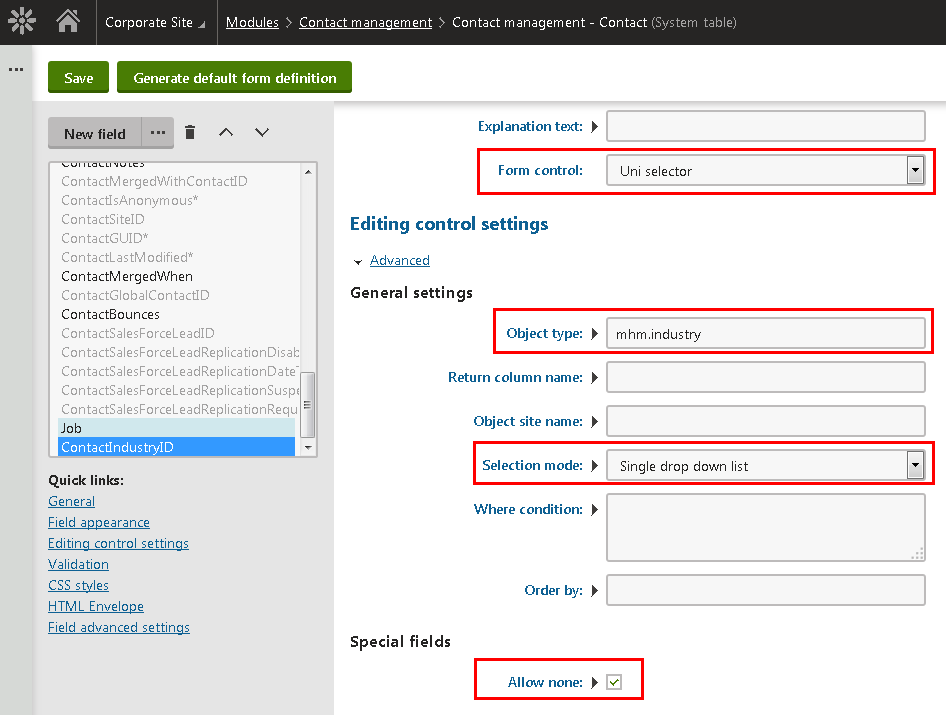The screenshot showcases a corporate website interface. At the top, a black band bears the label "Corporate site." Directly below, a menu bar features icons of a flower and a house, followed by the text "Corporate site," with pull-down modules labeled as "Contact Management" and "Contact System Table" underneath.

Below this menu, there are options to "Save," "Generate Default Form Definition," and a "New Field" button beside a trash can icon. Up and down arrows are present for navigating through selectable fields.

A section for field customization follows, where users can input various data, including "Explanation Test." This field is accompanied by "Form Control UNI Selector," which features a downward menu. 

Highlighted with a red rectangle are "Editing Control Settings" and "Advanced General Settings," indicating they are being modified. These sections include empty data fields for "Object Type," "Industry," "Return Column Name," "Object Site Name," and "Select Module." 

The single drop-down list under "Select Module," and the "Where Condition" and "Order By" fields, are also emphasized with red rectangles due to their empty states. The "Allow None" option is checked and similarly highlighted.